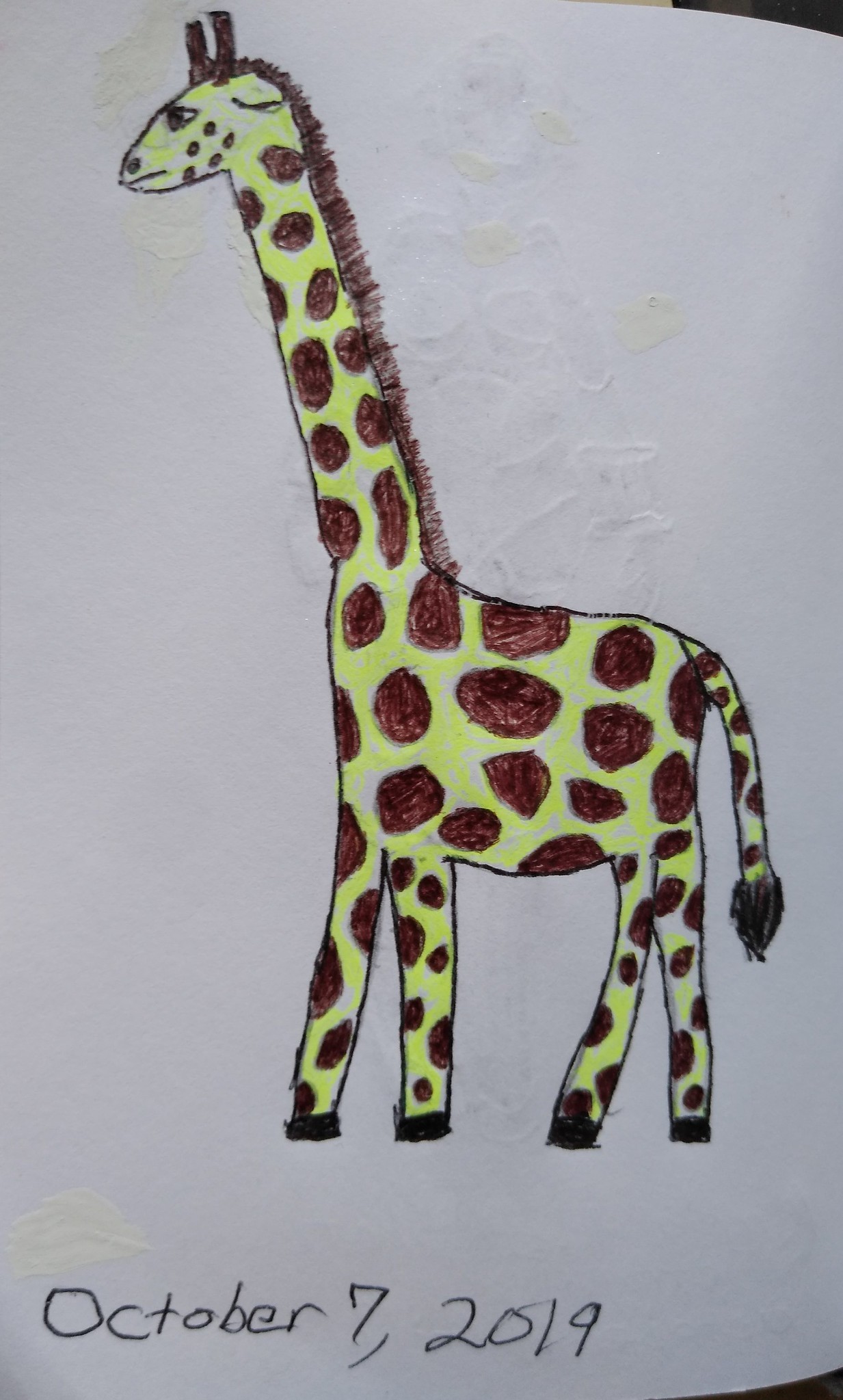This image is a close-up photo of a child’s drawing of a giraffe, sketched on a white piece of paper or a page of a sketchbook. The illustration is dated "October 7, 2019," written neatly in black pen at the bottom. The giraffe, facing left, is outlined in black ink and colored mainly with fluorescent yellow marker. It has distinct brown patches dotting its legs, body, tail, neck, and cheek. The giraffe’s legs end in black hooves, and its tail has a black, hairy tip. It features a brown mane running down the back of its long neck, brown ears, and brown, pointed ossicones (horns). The face shows intricate details with a serious, almost frowning expression, marked by small dots under its eye, and is finished with a black nose and a black line representing the mouth. The mixed media likely includes a combination of markers and colored pencils. The image hints at another drawing on the reverse side, although it is not visible.